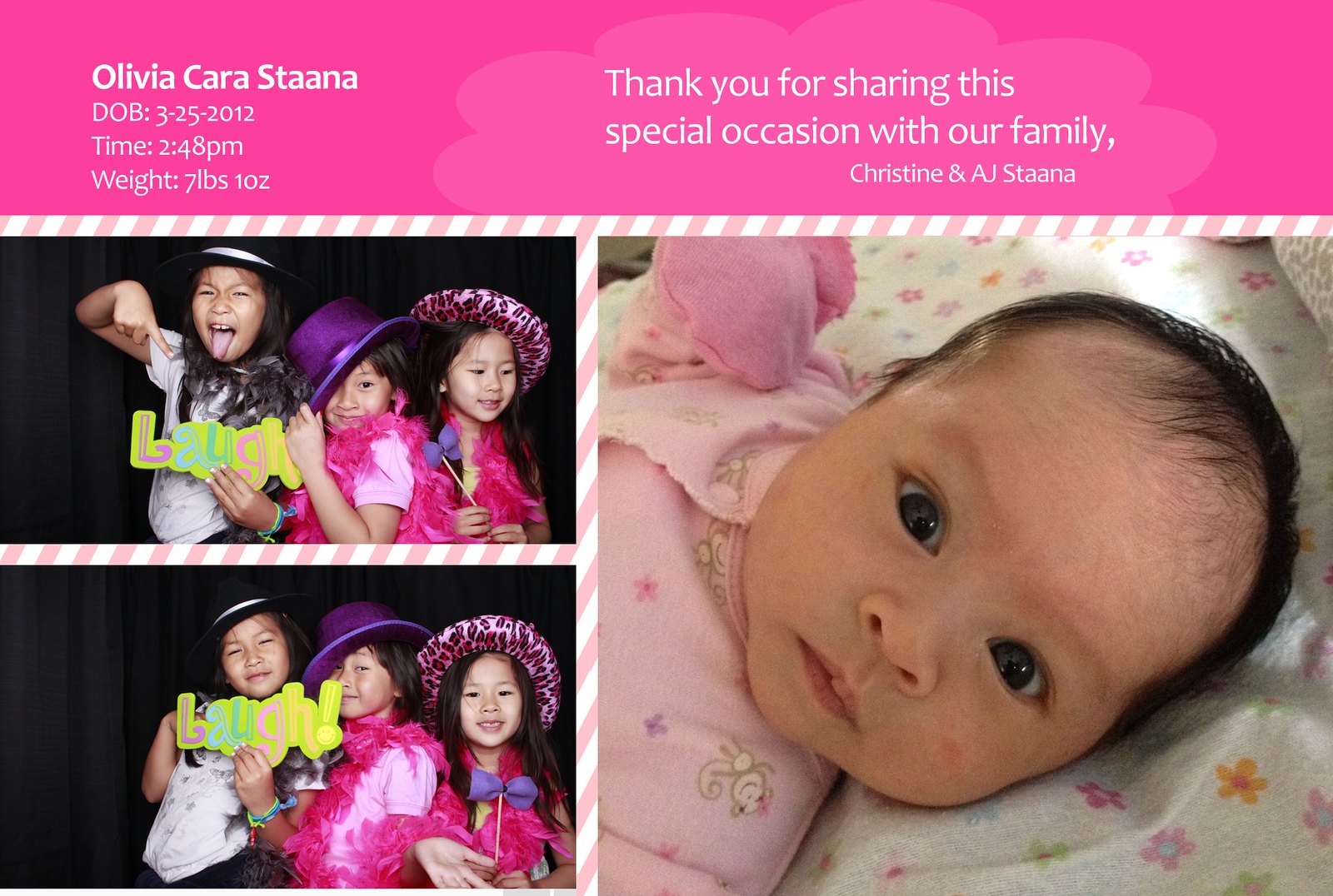This horizontally aligned rectangular thank-you card celebrates the birth of Olivia Karastana. The top quarter features a pink border with white text that reads: "Olivia Karastana, DOB: 3-25-2012, Time: 2:48 PM, Weight: 7 pounds, 10 ounces. Thank you for sharing this special occasion with our family, Christine and A.J. Stana." 

Below this, the card is divided into three sections. On the left side, two smaller horizontal images depict three young girls posing playfully in brightly colored outfits. The oldest girl wears a pink leopard print hat, and another girl wears a purple hat with the word "laugh" in multicolored letters.

The right side of the card holds a larger, close-up image of the newborn baby, Olivia, resting on a floral-patterned blanket. She wears pink baby clothes with floral and monkey patterns and has pink gloves. Olivia's eyes are open, and she stares adorably at the camera, with a hint of fine black hair visible on her head.

Striped white and pink borders separate the sections, enhancing the card's vibrant, celebratory design.